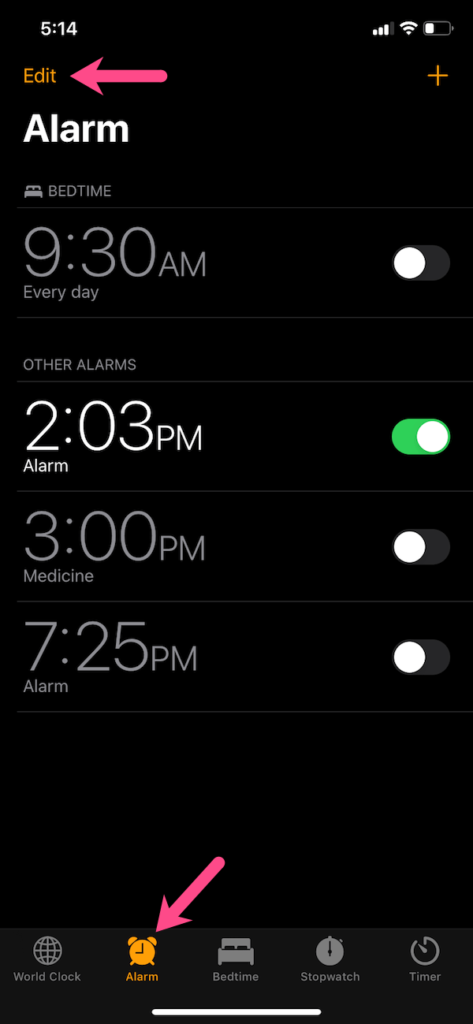The image showcases a smartphone screen displaying the alarm settings interface. At the top, crucial indicators such as the time (5:14), cellular signal bars, and the WiFi symbol are visible. Below these indicators, there is an "Edit" button highlighted by a pink arrow pointing towards it, suggesting user interaction. Also, an orange plus sign is featured, likely for adding new alarms.

On the screen, two main sections are present: "Alarm" and "Bedtime." The section labeled "Bedtime" includes an icon of a bed and a grayed-out notification stating "9:30 a.m. every day," which indicates the feature is currently turned off. Under "Other Alarms," a series of alarms are listed: one is set for 2:03 p.m. with a green active indicator, another for 3:00 p.m. labeled "Medicine" which is grayed out, and the last for 7:25 p.m., also inactive, labeled simply as "Alarm."

At the bottom of the screen, a navigation bar contains five icons: "World Clock," "Alarm" (highlighted in orange to indicate the page currently displayed), "Bedtime" with a bed icon, "Stopwatch" symbolized by a watch, and "Timer." Another pink arrow directs attention to the "Alarm" button at the bottom, likely guiding the user to this menu for modifying settings or creating new alarms. The overall design uses a black background with white numbers for clarity and readability.